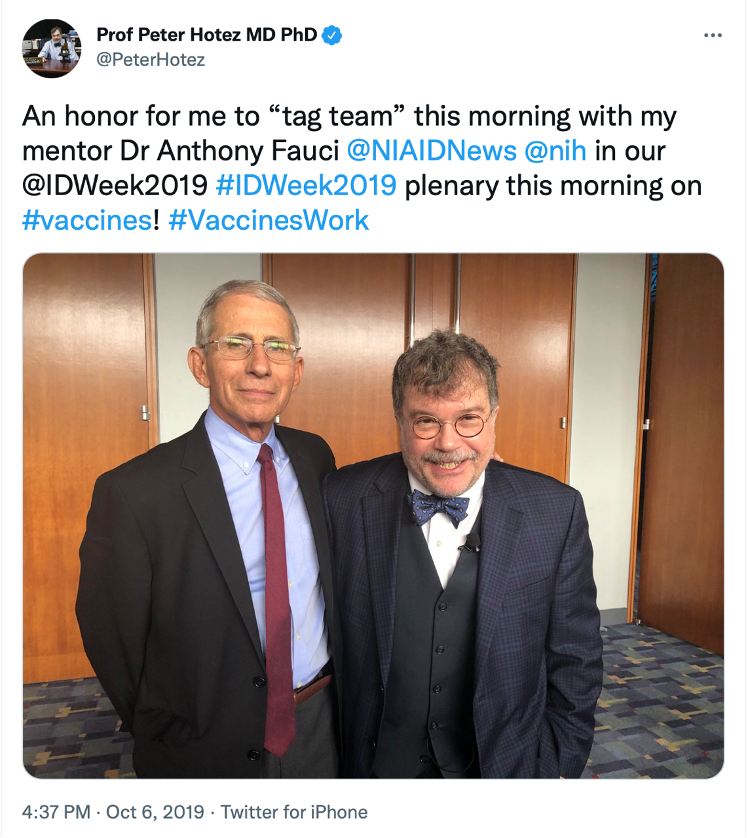The image depicts a Twitter post from Professor Peter Hotez, MD, PhD, posted at 4:37 PM on October 6, 2019, via Twitter for iPhone. The tweet, from his verified account (@PeterHotez), reads: "An honor for me to tag team this morning with my mentor, Dr. Anthony Fauci, @NIAIDnews at NIH, at our @IDWeek2019 plenary this morning on vaccines. #IDWeek2019 #VaccinesWork." 

In the accompanying photograph, Professor Peter Hotez stands on the right, attired in a blue Navy suit jacket, black vest, and blue bow tie. He has gray hair, circular glasses, and a mustache, and he is smiling. Dr. Anthony Fauci is on the left, wearing a blue shirt with a red tie, black jacket, gray hair, and glasses. The two are in a room featuring a carpet and brown doors. The header of the Twitter post shows Professor Hotez's profile picture in the top left corner along with his name and a blue verification check mark.